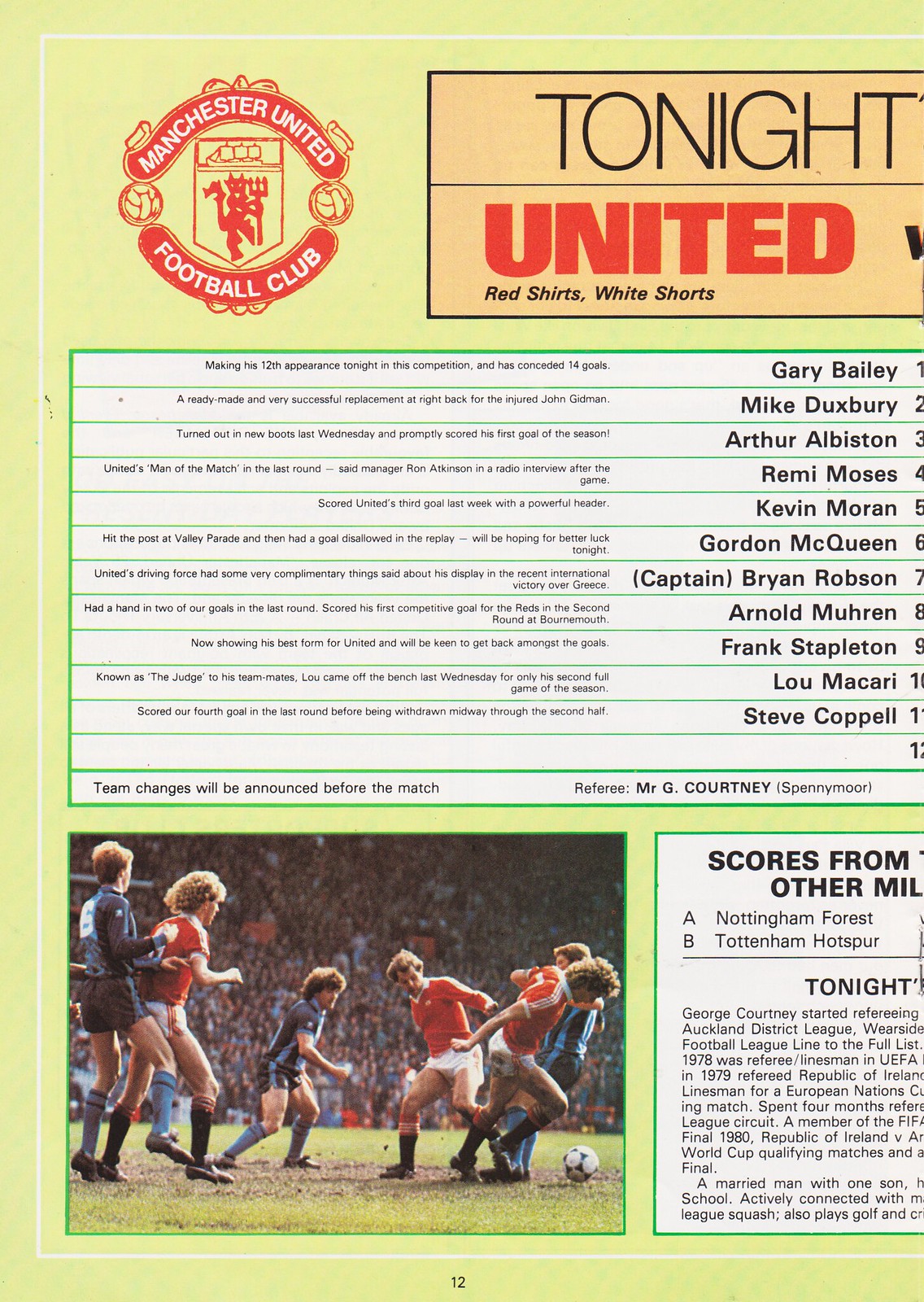The image appears to be a detailed, partially truncated poster or page from a sports magazine, primarily in a light lemon yellow background. Prominently featured in the upper left is the Manchester United Football Club logo in red and orange, accompanied by a couple of footballs in a banner style. Adjacent to this, the headline reads, “Tonight, United,” with additional text indicating "red shirts, white shorts," although part of the headline is cut off, as is the right side of the image.

Central to the poster on a white background is the lineup for Manchester United. It lists eleven players with their assigned numbers and brief highlights of their recent performances. The players include:
1. Gary Bailey: Making his 12th appearance, having conceded 14 goals.
2. Mike Duxbury: Replacement at right back, scored his first season's goal recently.
3. Arthur Albiston: Man of the match as per Manager Ron Atkinson.
4. Remy Moses: Scored United’s third goal last week with a powerful header.
5. Kevin Moran: Had a goal disallowed previously, hoping for better luck.
6. Gordon McQueen: Praised for his display in an international victory.
7. Captain Brian Robson: Contributed to two goals in the last round.
8. Arnold Muhren: Exhibiting his best form, keen to score.
9. Frank Stapleton: Known as "the judge," recently made his second full game appearance.
10. Lou Macari: Scored in the last round before being substituted.
11. Steve Coppell.
A placeholder for player number 12 indicates potential team changes to be announced before the match, and it mentions referee Mr. G Courtney.

In the lower left section, there's an action-packed image of players donning red shirts with white shorts vs. blue shirts with blue shorts in a football match. The pitch is crowded with a cheering audience in the background.

To the right of this image, there is a partially visible section labeled "Scores from Other Mill," listing incomplete text about teams like Nottingham Forest and Tottenham Hotspur. Additional information pertains to George Courtney’s refereeing history, though it’s partially obscured.

Overall, the imagery combines both promotional and informational elements regarding Manchester United's lineup and their ongoing match activities.